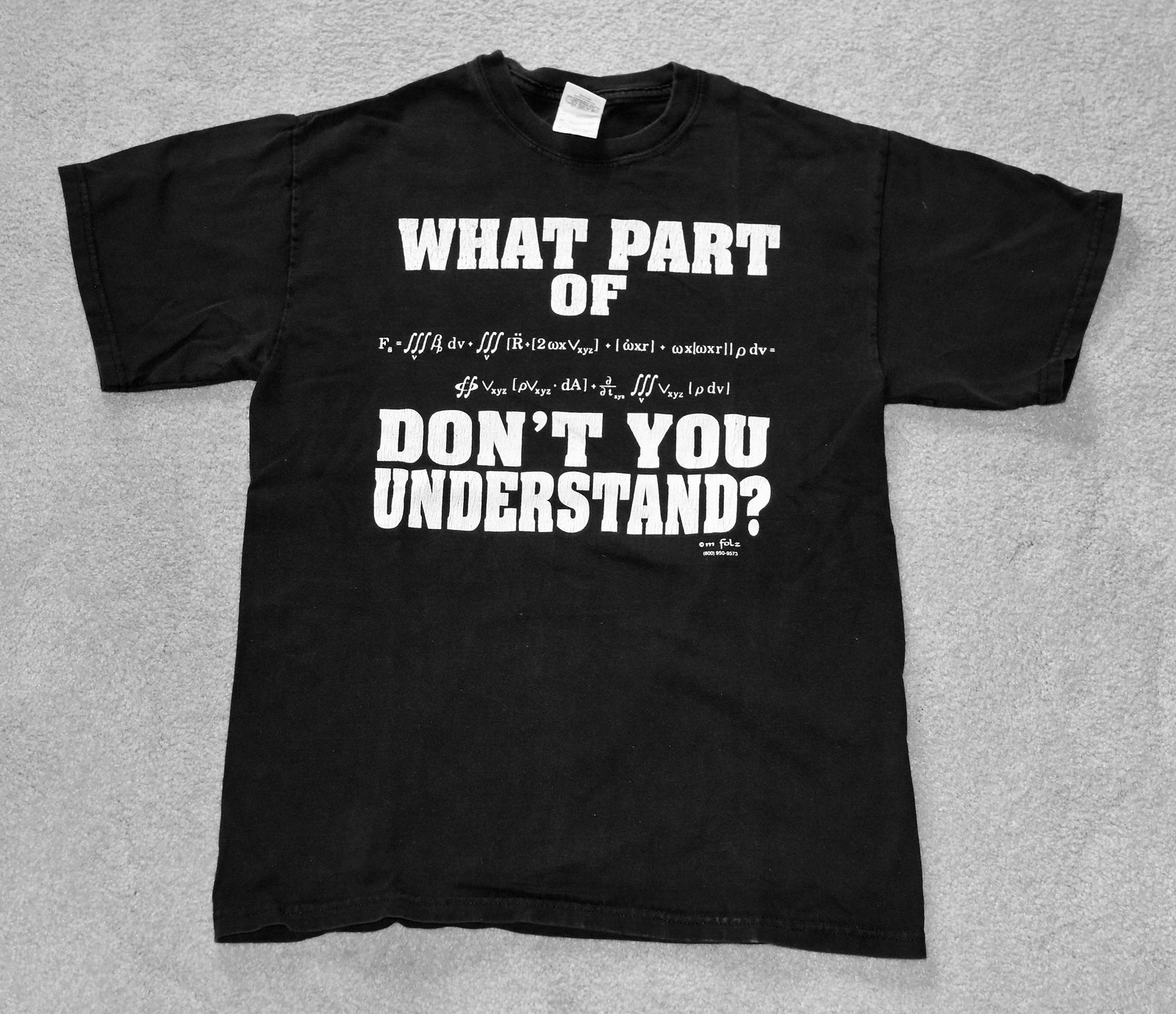The image displays a black short-sleeved t-shirt, meticulously laid flat with arms straight out, on a textured surface that appears to be a fluffy, purple carpet. The carpet might also seem light gray depending on the perspective. The focus of the t-shirt is the bold, white block text across the front. The top line prominently reads "WHAT PART OF" in capital letters, followed by a complex mathematical formula spanning two lines in the middle. Below the formula, another line of bold, white text reads "DON'T YOU UNDERSTAND?" with a question mark. There is also a small, unreadable watermark or copyright notice at the bottom right under the 'D' and question mark. A white tag is visible at the top collar of the shirt, which is slightly flipped, obscuring any further details. The overall setup and high-quality visualization suggest this might be an image intended for an online store.